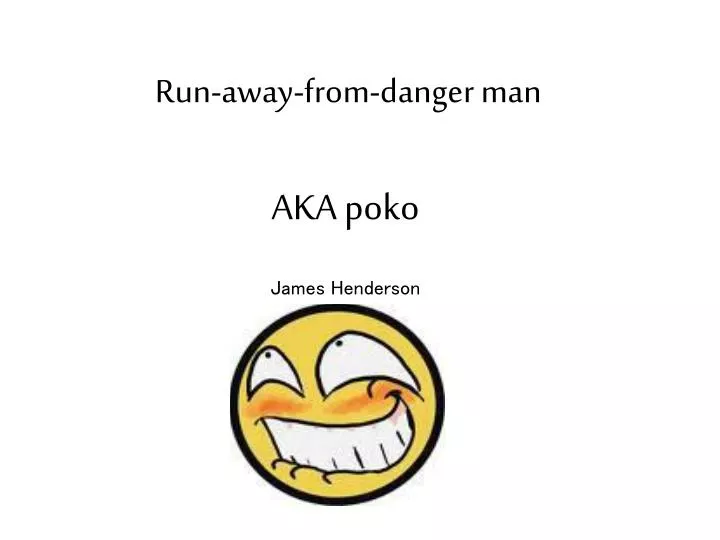The image features a stark white background with black text at the top that reads, "Run Away From Danger Man." Beneath this, in all caps, it says "AKA Poco," followed by the name "James Henderson" in smaller font. Below the text is a heavily stylized yellow emoji. The emoji has a black outline and its eyes, filled with white and black pupils, look upwards and leftwards. It has a wide, toothy grin, with its lower lip tucked under its upper teeth, mimicking a sly, amused expression. The emoji features an orange blush on its cheeks, accentuating its mischievous grin, reminiscent of the Grinch's smile.